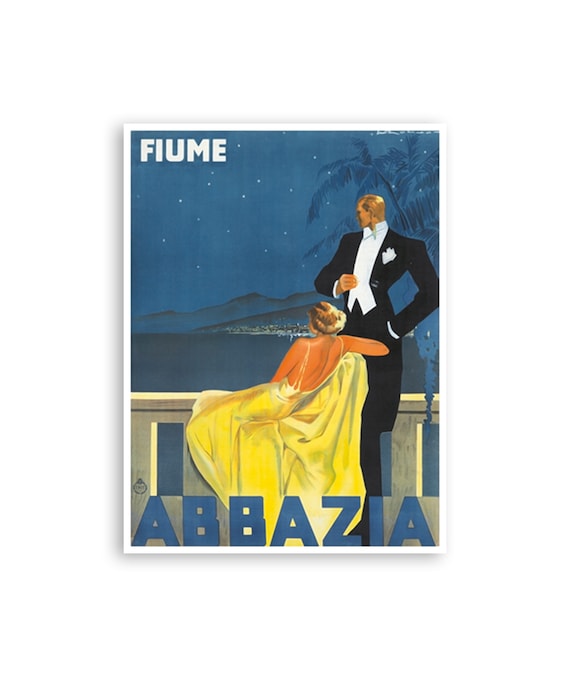This detailed image, reminiscent of an advertisement or a magazine cover, depicts a picturesque night scene framed within a white border, featuring elements of Art Deco illustration. The background is a rich dark blue, dotted with stars, suggesting a serene, starlit night. In the image, a blonde woman, dressed in a stunning, backless, golden-yellow dress, sits with her legs draped over the stone railing of a balcony. Her gaze is directed towards the tranquil expanse of the sea, which is dotted with distant lights suggesting a coastal village or town. 

Beside her stands a man with a striking, statuesque appearance; his impeccably polished bronze-like head gleams. He is elegantly attired in a black three-piece suit, consisting of a black jacket, matching pants, a white vest, and a white pocket square. The man, too, looks out over the railing, perhaps lost in thought as he takes in the view. 

A silhouetted palm tree subtly adorns the right-hand side of the image, adding a touch of exotic elegance. The stone railing, against which the man stands and over which the woman drapes her legs, punctuates the scene with its geometric cutouts, revealing glimpses of the sea below. 

Text overlays punctuate the image: the name "FIUME" in bold white letters at the top, and "ABBAZIA" in large blue letters across the bottom, anchoring the visual narrative of this captivating, poster-like illustration.